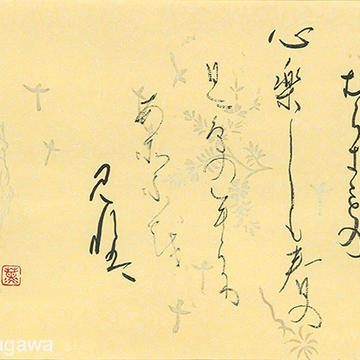The image features a yellow or beige colored background with an array of hastily scribbled, black ink writings. These inscriptions are difficult to decipher, potentially challenging even for those who read Chinese due to their rapid, almost careless execution. Dominating the bottom left corner is a noticeable red stamp bearing a Chinese character. Surrounding this stamp are several vertical columns of writing, each varying in darkness and length. The rightmost column is the darkest and extends the furthest, while the center and left columns are lighter and shorter. Adding an intriguing layer to the chaotic text are two faint, light-colored crosses positioned above the red stamp. The overall impression is one of haste and randomness, with minimal attention to readability or form.